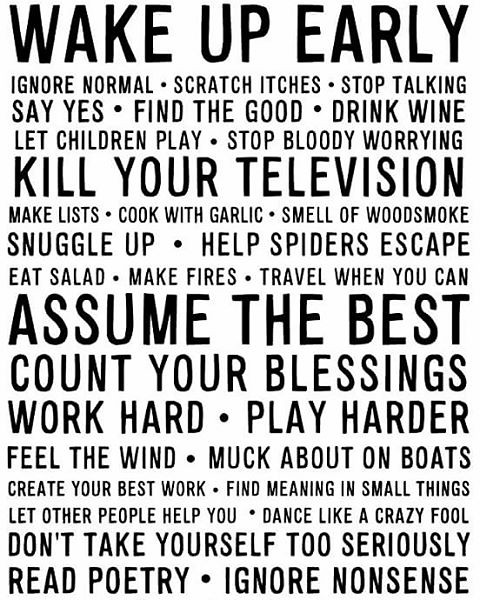The image consists of a simple white background with black type, creating a stark yet impactful visual. The background remains entirely plain and empty, emphasizing the significance of the text that spans the entire image. The text is presented in all caps, with varying sizes to highlight certain phrases. At the top, in bold text, it starts with "WAKE UP EARLY." Following this, in regular size, it continues: "IGNORE NORMAL, SCRATCH ITCHES, STOP TALKING, SAY YES, FIND THE GOOD, DRINK WINE, LET CHILDREN PLAY, STOP BLOODY WORRYING." A larger type then emphasizes the phrase "KILL YOUR TELEVISION." In smaller type below, it lists: "MAKE LISTS, COOK WITH GARLIC, SMELL OF WOOD SMOKE, SNUGGLE UP, HELP SPIDERS ESCAPE, EAT SALAD, MAKE FIRES, TRAVEL WHEN YOU CAN." The next highlighted phrase in larger type reads: "ASSUME THE BEST, COUNT YOUR BLESSINGS, WORK HARD, PLAY HARDER." This is followed by slightly smaller type: "FEEL THE WIND, MUCK ABOUT ON BOATS, CREATE YOUR BEST WORK, FIND MEANING IN SMALL THINGS, LET OTHER PEOPLE HELP YOU, DANCE LIKE A CRAZY FOOL, DON'T TAKE YOURSELF TOO SERIOUSLY, READ POETRY, IGNORE NONSENSE." The careful arrangement of the text and varying font sizes emphasize key messages, creating a motivational and thoughtfully designed visual.